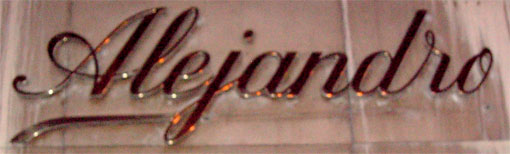The image features a name, "Alejandro," written in an elegant cursive script against a pinkish background. The background lightens towards the left and right edges, with the right side having more of the lighter pink hue. It appears to be composed of tile-like bars, possibly suggesting a decorative or structured surface. The name "Alejandro" is crafted in a striking blend of brown with orange and white sparkles, giving it a glittering, metallic appearance. The script includes a distinctive extension from the letter 'J' that reaches toward the left-hand corner, adding a unique artistic touch. This ornate lettering could be indicative of a nameplate for a restaurant or club, evoking a sophisticated and possibly upscale ambiance.